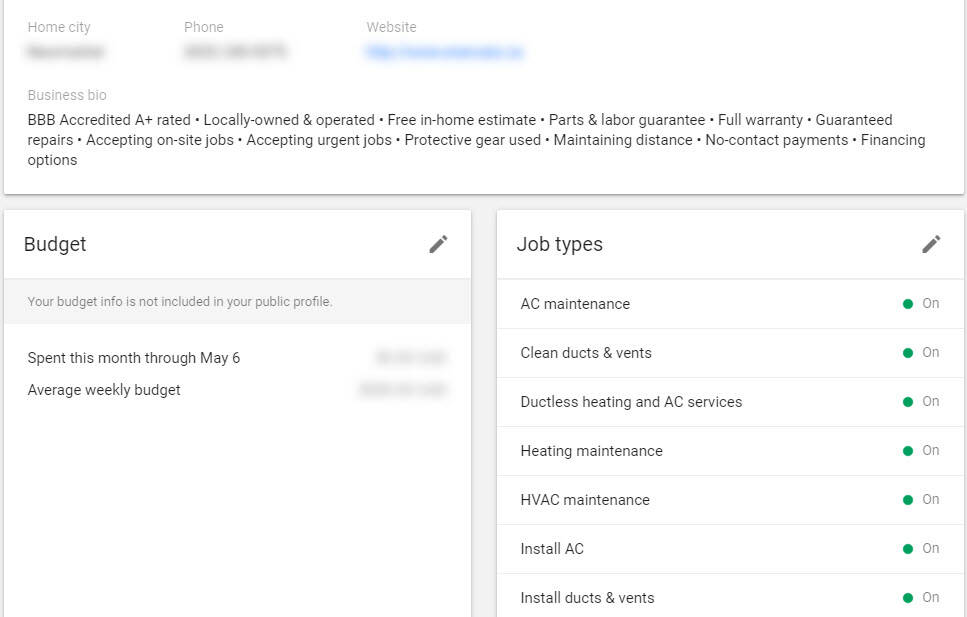The image portrays a segmented user interface, predominantly featuring rectangles with varied outlines and filled sections. Starting at the top, there's a partially outlined rectangular section in grey, lacking the outline on the upper edge. Within this section, the background is white. The top header contains greyed-out text fields labeled "Home City," "Phone," and "Website." Below that, there is a segment titled "Business Bio" with accompanying information.

To the left, another rectangular section is outlined in grey on the top and sides but is open at the bottom. This section is labeled "Budget" and includes a pencil icon on the right side, possibly indicating an edit function. Inside, there is text too small to read, followed by greyed-out text reading "Spent this month through May 6th" and "Average weekly budget."

Next, there is another similarly styled rectangular section labeled "Job Types," also featuring a pencil icon on the right. Within this section, it lists various job types each followed by a green dot and the word "On", indicating active status. The listed job types are:
- "AC Maintenance"
- "Clean ducts and vents"
- "Ductless heating and AC services"
- "Heating Maintenance"
- "HVAC Maintenance"
- "Install AC"
- "Install ducts and vents"